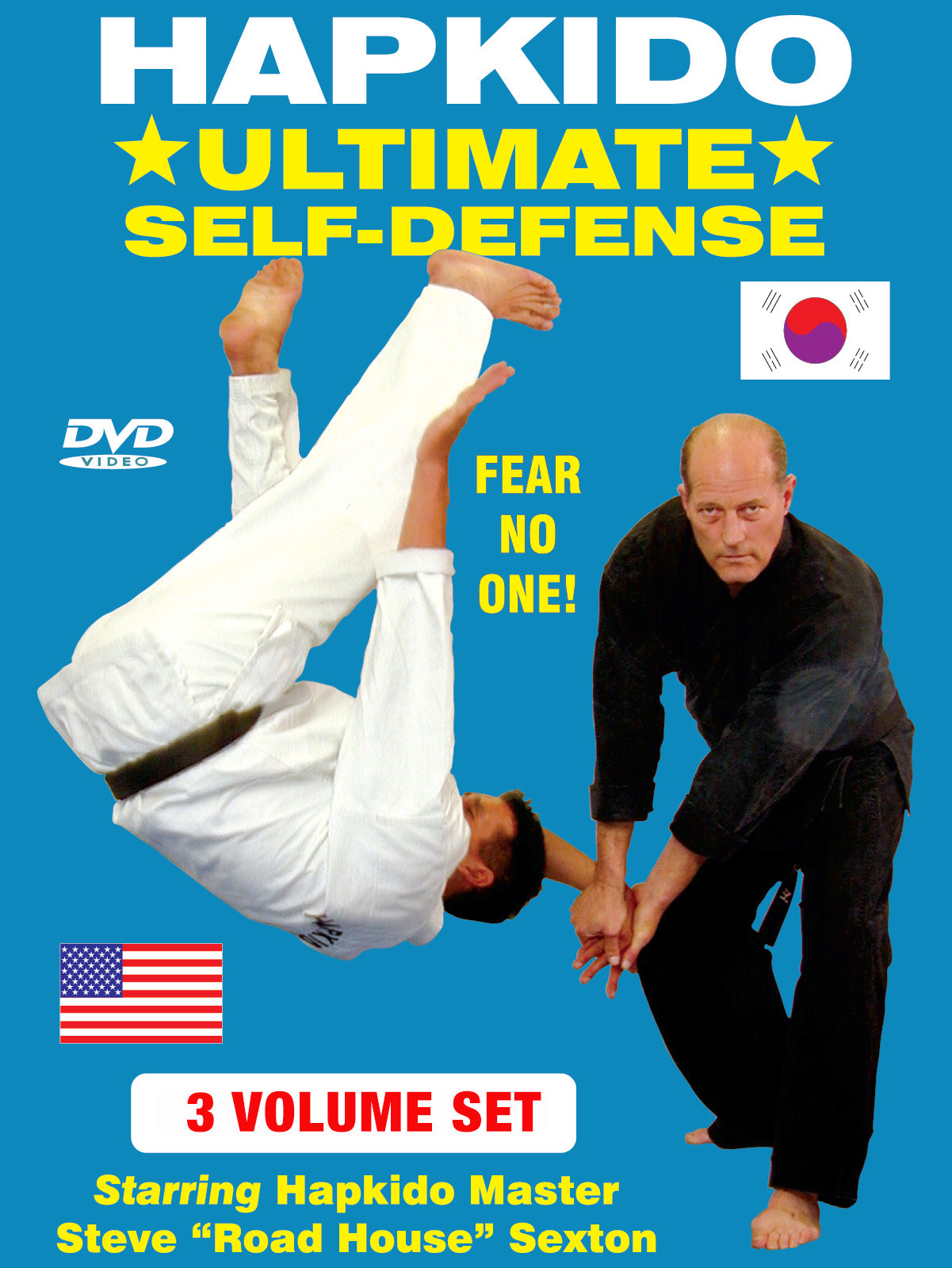This image is an advertisement for a self-defense DVD set titled "Hapkido: Ultimate Self-Defense." At the top of the image, in bold white text, is "Hap Ki Do," and in bold yellow text, "Ultimate Self-Defense," both overlaid on a blue background. To the right of these words, there is a flag resembling the yin-yang symbol but in red and purple instead of black and white. Below this, the words "DVD Video" are displayed prominently. The focal point of the image shows two men performing a self-defense maneuver: a man in a black robe pinning down and flipping a man in a white robe with a black belt. The caption "Fear No One" is positioned next to the individual in mid-flip. At the bottom left corner, text reads "Three Volume Set" in a white rectangle with red lettering, and it mentions that the set stars "Hapkido Master Steve 'Roadhouse' Sexton." Additionally, an American flag is depicted next to the text.